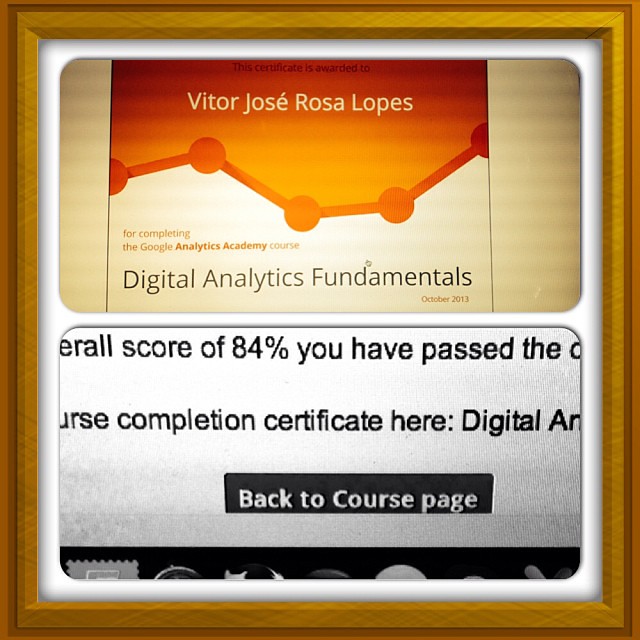The image showcases a certificate displayed within a two-sectioned wood frame. The top section features an orange background with the name "Vitor Jose Rosa Lopez" prominently displayed in a rounded rectangle. Below this, there is a filled line graph with white underneath that reads "Digital Analytics Fundamentals" in black text. This indicates that the certificate is for completing the Google Analytics Academy course in October 2013. The bottom section of the frame contains text that is partially cut off, but it likely includes an overall score of 84%, confirming that Vitor Jose Rosa Lopez has passed the course. The entire certificate appears to be a black and white printout of a web page, neatly inset into the brown frame.